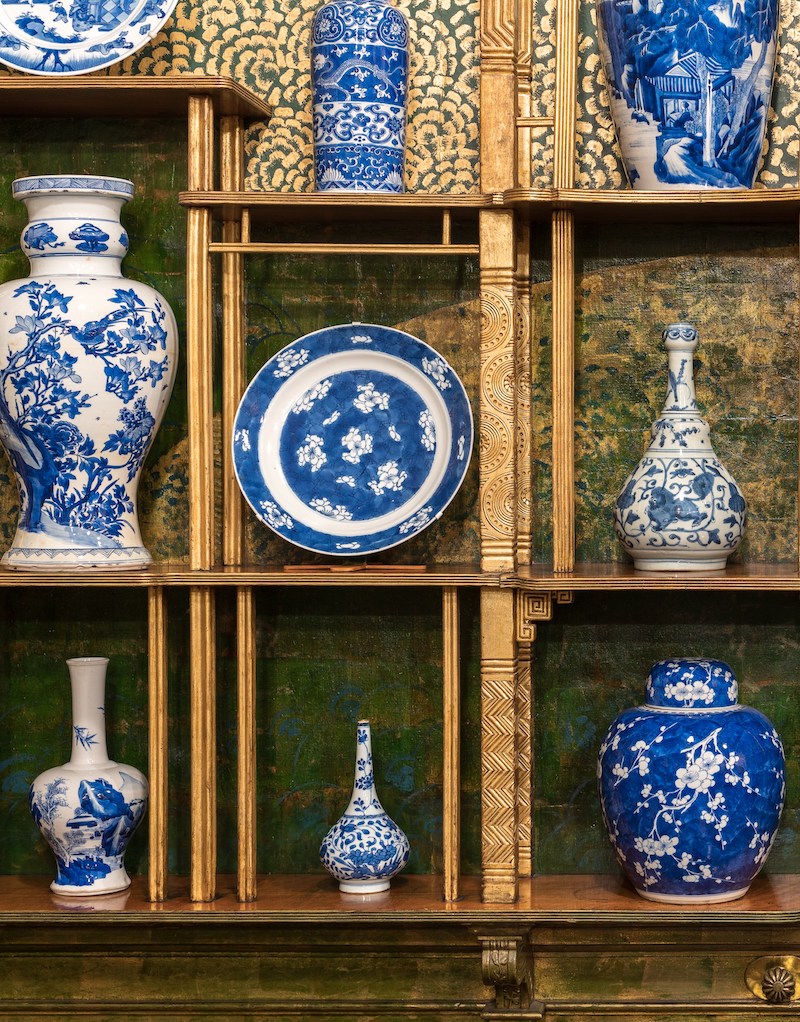The photograph captures an indoor scene of a meticulously designed shelving unit against a creatively decorated wall. The shelving unit features thin wooden shelves, separated by golden columns with intricate patterns, giving a royal aesthetic. The backdrop transitions from a green base with gold petal designs at the top, to a subtle interspersing of gold and blue towards the bottom. The shelves house an elegant collection of ceramic pottery, predominantly blue and white, exuding a chinoiserie style. The top-left corner displays a plate, accompanied by variously sized vases extending to the right. The middle row includes another plate flanked by a vase and a bottle. The bottom shelf showcases a long-necked vase, a narrow-topped flower vase, and a capped urn, all of which contribute to the refined and classy appearance of the arrangement. This visually arresting display suggests a shop or gallery setting, showcasing artifacts with artistic precision.